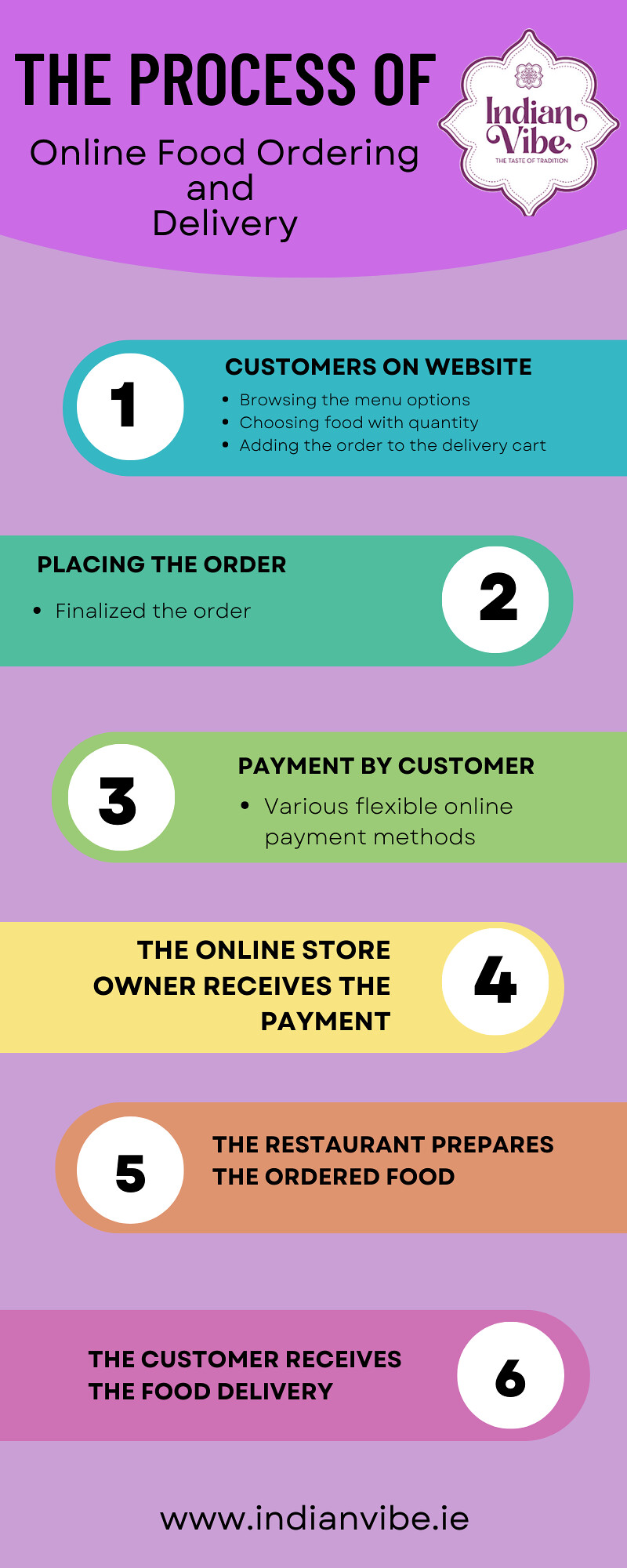The image is a detailed advertisement from Indian Vibe, elucidating the process of online food ordering and delivery. Dominated by a purple background, the advertisement features the Indian Vibe logo situated in the top right corner. The main content comprises six distinct, colored horizontal lines, each outlining a specific step in the ordering process. The steps are as follows: Step one, in blue, indicates "Customers on website". Step two, in dark green, covers "Placing the order". Step three, in light green, details "Payment by customer", highlighting various flexible online payment methods. Step four, in yellow, shows "The online store owner receives the payment". Step five, in orange, describes "The restaurant prepares the ordered food", and step six, in pink, concludes with "The customer receives the food delivery". At the bottom of the image, the website URL "www.indianvibe.ie" is prominently displayed, guiding customers to further information and services offered by the restaurant. The advertisement effectively educates its audience on the seamless process of online ordering from Indian Vibe.